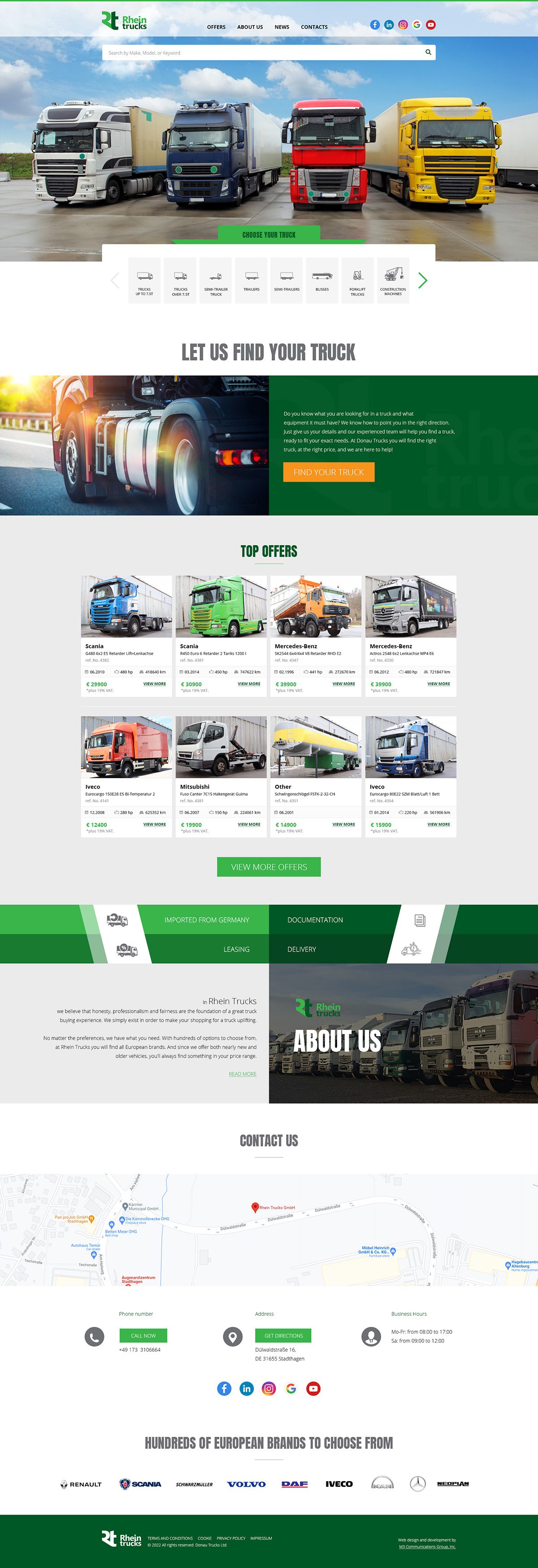The image displays the homepage of a truck-related website. The logo in the top left corner includes the word "trucks," and adjacent to it are tabs and links to various social media pages like Facebook and Instagram. A prominent white search bar stands out at the top of the page.

Below the header, there is a visually striking image featuring four trucks: one white, one blue, one red, and one yellow. This section transitions into a green area interspersed with gray boxes containing various logos, accompanied by the text "Let us find your truck" in gray. To the left of this, a picture showcases the wheels of a truck, alongside a green box with white text and a prominent yellow button.

Further down, the "Top Offers" section is displayed, featuring multiple images of trucks organized into two rows and four columns. The trucks come in various colors, including green, orange, blue, white, and red. Another green area follows, containing several links.

The section labeled "About Us" is located on the right, with a paragraph of explanatory text in gray on the left. Beneath this, the "Contact Us" section includes a map and several green buttons at the bottom. The page concludes with a statement, "Hundreds of European brands to choose from," showcased alongside logos of multiple brands.